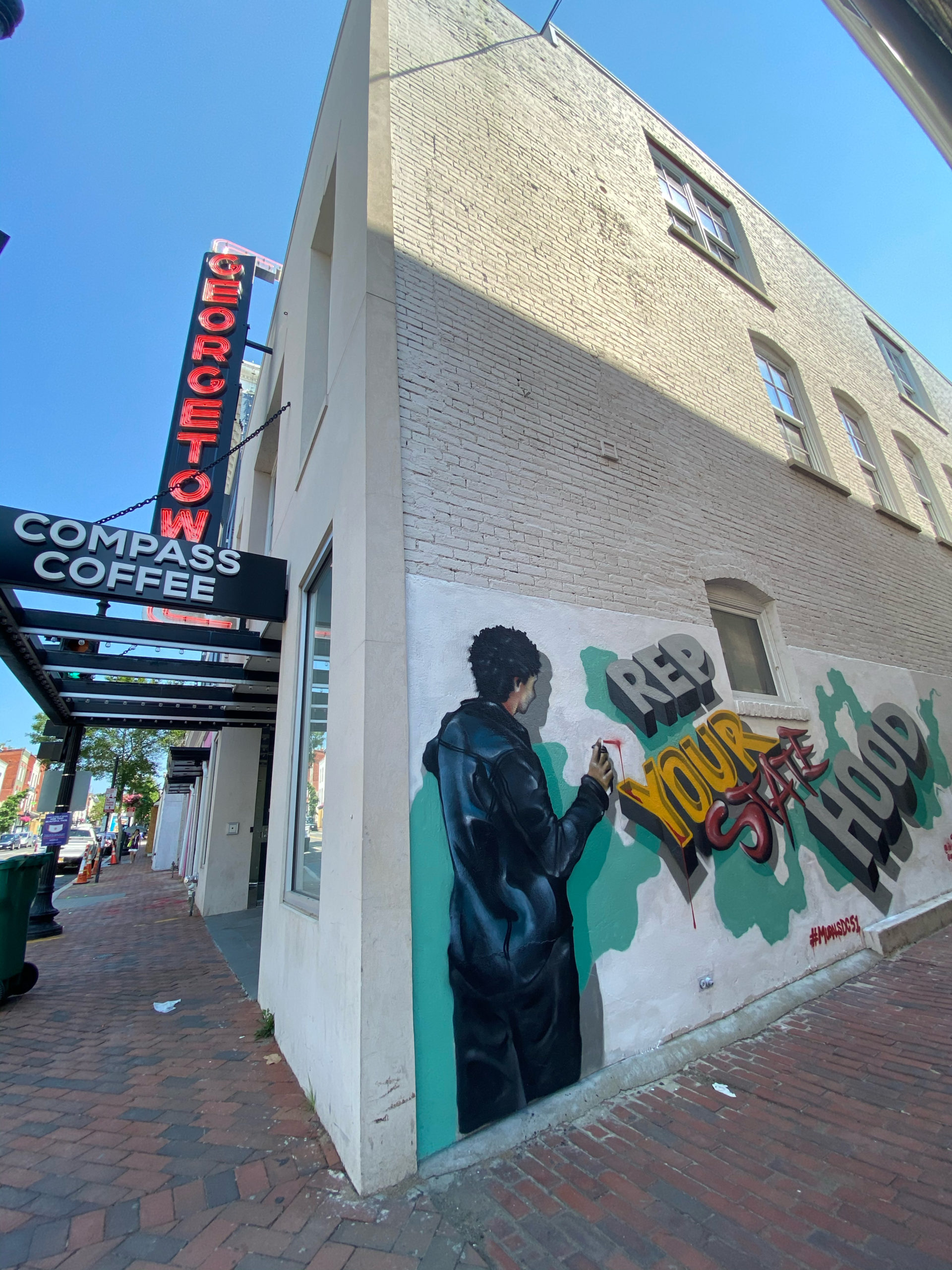The image portrays a stucco building with white bricks and multiple windows, set against a clear blue sky. At the top of the building, a sign reads "Georgetown Compass Coffee," though the letter "N" is partially obscured. A central feature of the scene is a piece of graffiti spanning a corner of the wall. This graffiti, which reads "rep your statehood," depicts a black individual in a black trench coat holding a spray paint can, seemingly in the act of creating the artwork. The building’s lower and upper levels have several glass-pane windows, adding to the urban feel. The sidewalk in front is composed of red bricks, contributing to the contrasting textures and colors in this outdoor setting that captures a slice of city life, potentially in a more neglected area.